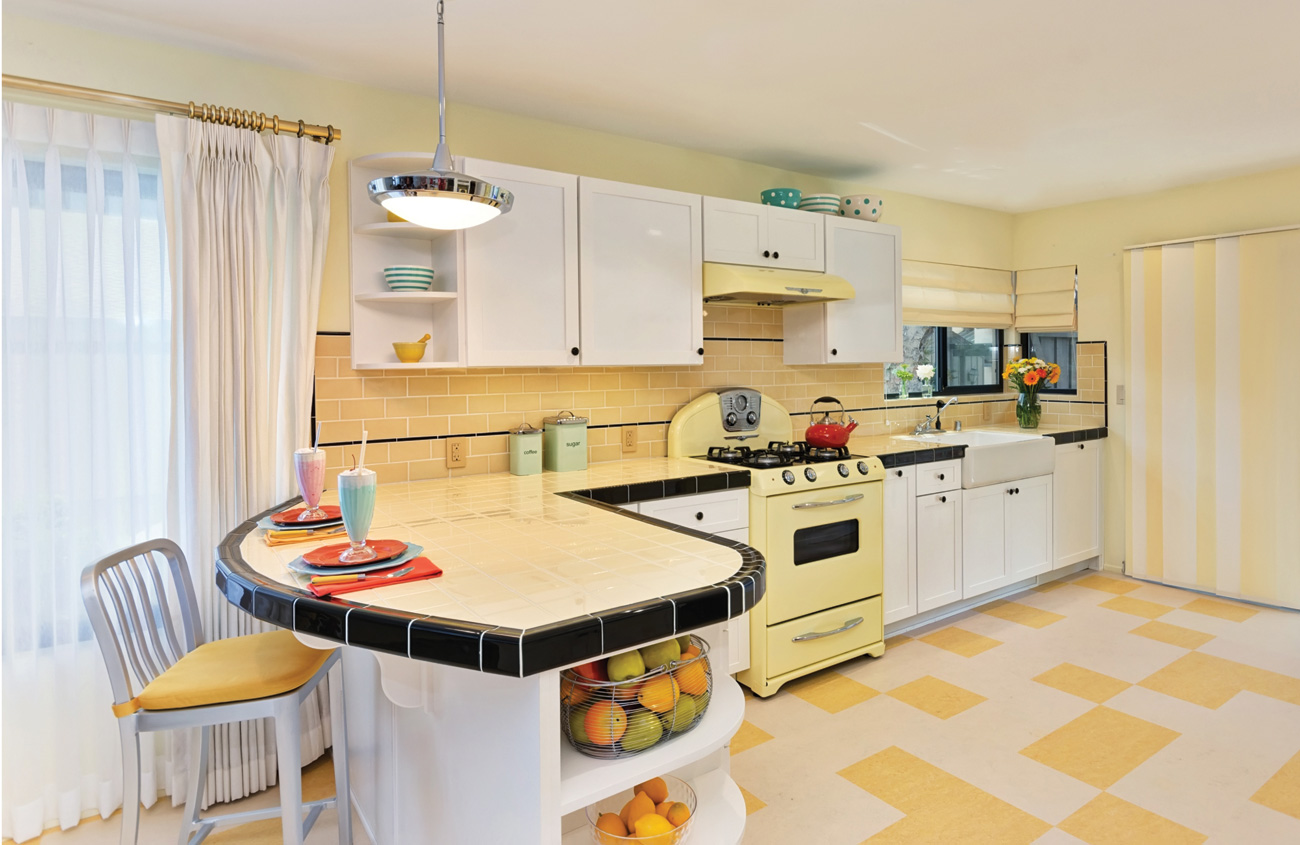This vivid, retro-style kitchen captures the charm of a bygone era with a delightful mix of vibrant colors and classic design elements. Dominating the center is a yellow stove with a matching yellow hood, accompanied by a striking red kettle. Surrounding the stove is a yellow countertop with black trim that forms an L-shape, adding a stylish twist. The cabinets above and below the countertop are pristine white, providing a fresh and clean look. The brick-patterned yellow walls add a warm touch, contrasting beautifully with the white ceiling.

To the right of the stove, a sink with a sleek faucet is nestled beneath a large window adorned with translucent white curtains, and a vibrant bouquet of flowers brings a touch of nature indoors. A sidewall on the right features a big yellow and white patterned door, enhancing the nostalgic feel of the space. Towards the bottom left, a modern stool with a yellow cushion underpins the retro aesthetic.

Above the milkshakes on the left side of the countertop, a bright light casts a warm glow, while white shelves and cabinets provide ample storage. The shelves are thoughtfully decorated with bowls, plates, and utensils. Two glass cups filled with colorful milkshakes and topped with straws rest invitingly on plates with napkins and spoons. Below the countertop, additional cabinets host a selection of fruits and kitchen essentials.

Adding to the lively atmosphere is a curving yellow-and-brown tiled floor, harmonizing perfectly with the overall color scheme. Completing the picture, the left side of the kitchen boasts a large window with a white curtain pulled to the side on a golden rod, further enhancing the airy and spacious feel of this lovingly designed retro kitchen.